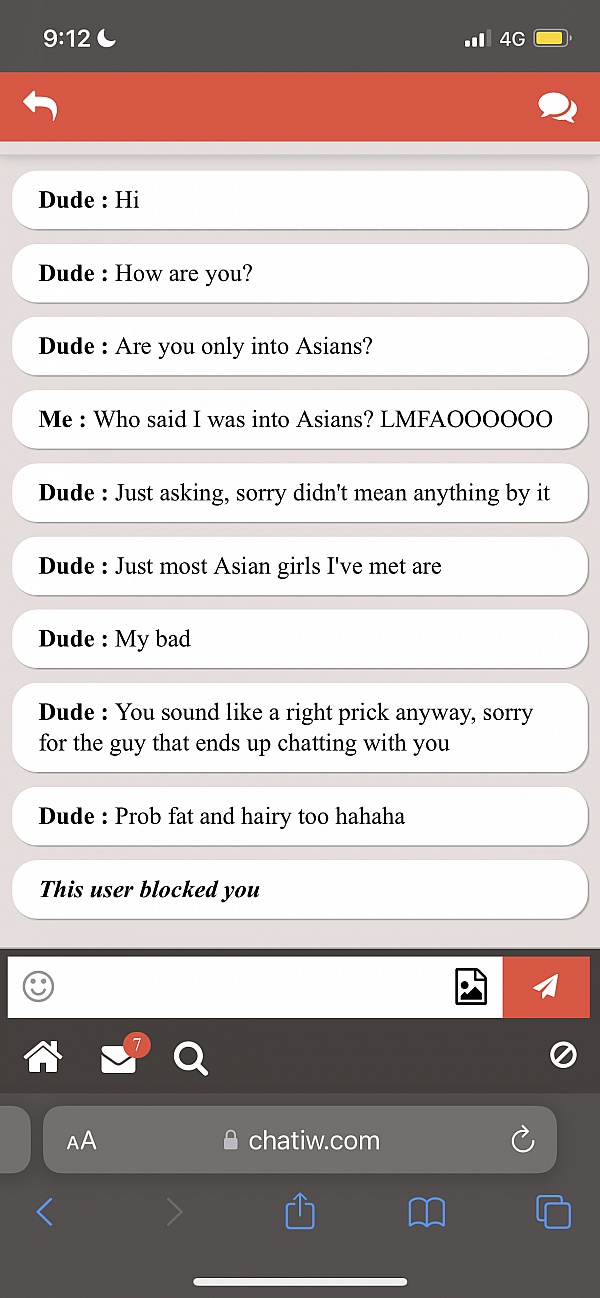**Detailed Caption:**

This color portrait-format screenshot, captured at 9:12, displays the home screen of a smartphone. A crescent moon icon is situated beside the time, which is often indicative of the device being in 'Do Not Disturb' mode rather than indicating lunar phases or AM/PM status. The phone shows strong connectivity with three out of four reception bars and indicates the user is connected to a 4G network. The battery icon suggests the device is almost fully charged.

The focus of the screenshot is a webpage—chatiw.com, presumable a chat website. The ongoing conversation displayed is a text thread between two users, identified as "Dude" and "Me" (the phone's user). The exchange is as follows:

- **Dude:** "Hi, how are you? Are you only into Asians?"
- **Me:** "Who said I was into Asians? LMFAO."
- **Dude:** "Just asking, sorry didn't mean anything by it. Just most Asian girls I've met are, my bad. You sound like a right prick anyway, sorry for the guy that ends up chatting with you. Probably fat and hairy too, ha ha ha."

The conversation concludes with a notification indicating that "this user blocked you," signaling that the phone's user has blocked "Dude."